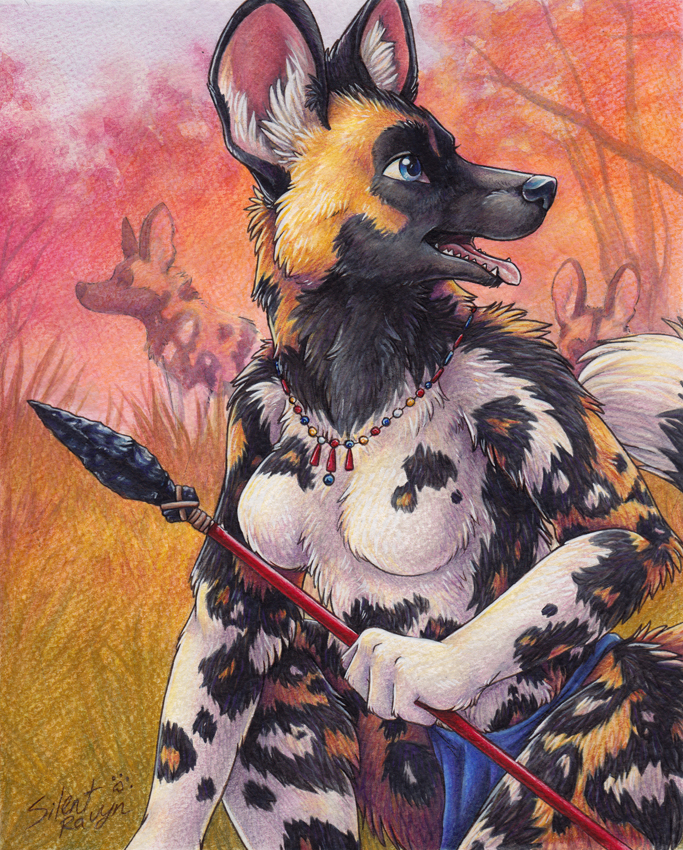The image appears to be a highly detailed colored pencil drawing depicting an anthropomorphic female creature, a blend of hyena and human characteristics. The central figure, a hyena woman, is crouching on the ground with her body oriented toward the left side of the image while her head is turned back, peering to the right with striking blue eyes and an open mouth. Her hyena face transitions into a body that, while largely hyena-like, includes human-like breasts adorned with a red, blue, and yellow necklace. In her left hand, she grips a spear with a distinct black stone tip and a red handle. The background features a field adjacent to a forest, populated by several other hyenas or wolf-like creatures. The scene is bathed in warm hues of orange and red, suggesting a sunset ambiance, although the precise details remain indistinct behind the central figure.